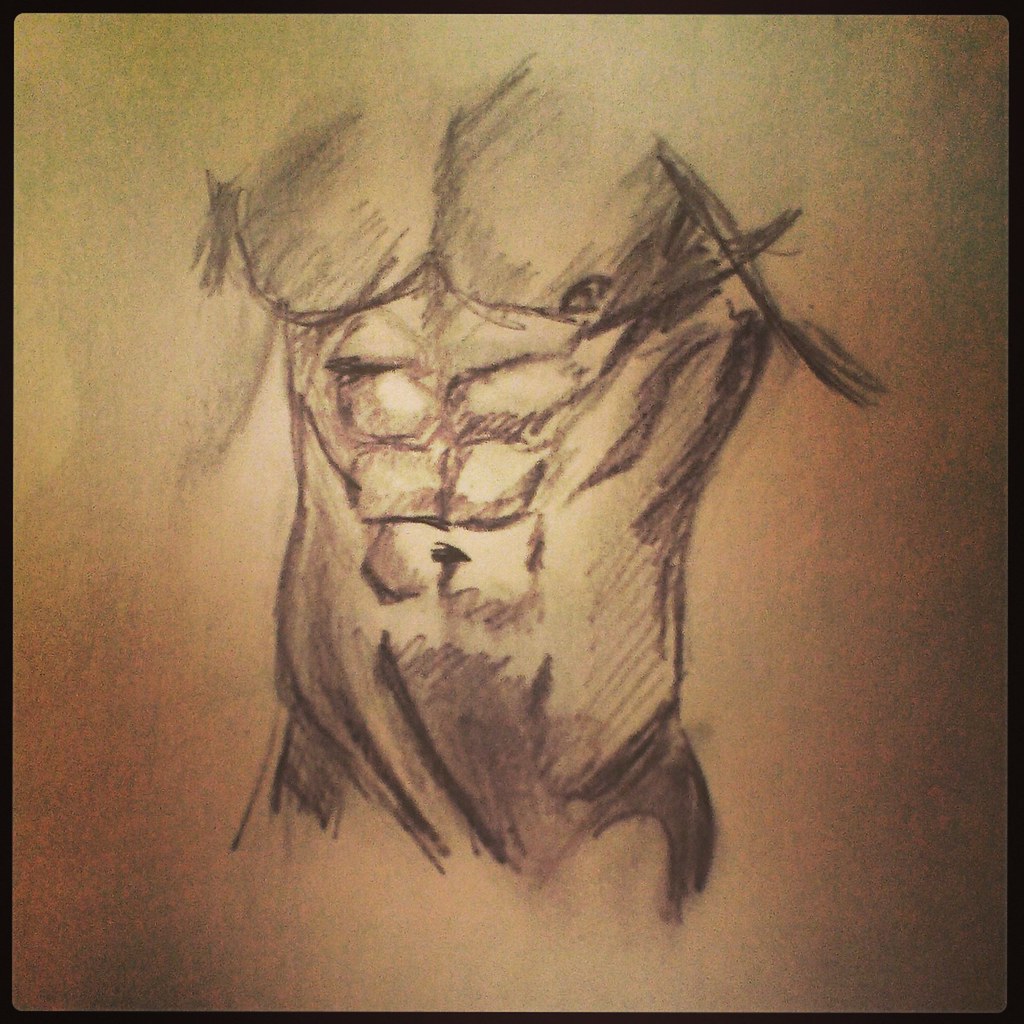The image is a photograph of a pencil or charcoal sketch depicting a male torso from the chest down to the hips. The sketch is highly detailed in some areas, such as the well-defined pectoral muscles and pronounced six-pack abs, highlighted with heavy, scribbly sketch marks. The drawing includes the inguinal V-shape and a roughly sketched navel. Broad lines and careful shading accentuate the musculature, while a faint outline suggests the collarbone and portions of the shoulders, though no head, arms, or legs are present. The sketch is bordered in black, and it is rendered on paper that appears to have a light brown hue with tan and white tones.